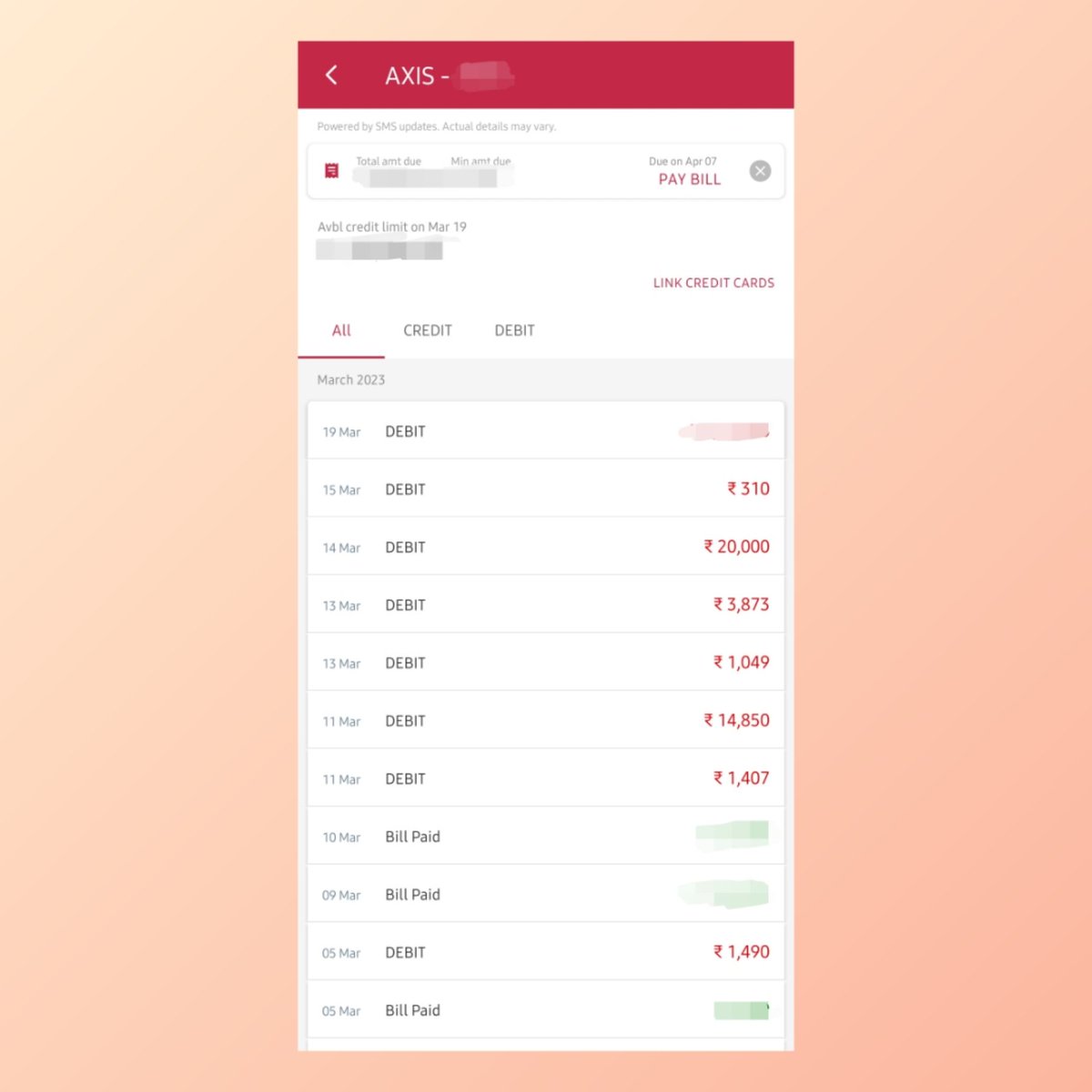This image appears to be a screenshot taken from a mobile phone, overlaid on a large pink background. The pink background extends approximately half an inch on the top and bottom, and about two inches on the left and right sides of the centered screenshot. The screenshot itself is rectangular, typical of a phone display.

Within the screenshot, the top segment—about an inch in height—is dark pink. On the left side of this dark pink area, there is a white greater-than sign (>) pointing to the left. Next to it, in all-capital white letters, is the text "8XIS-," followed by a blurred-out word.

Below this dark pink section, the background turns white. In the top-left corner, it states "powered by SMS updates." Below that line, a rectangle contains two key pieces of information: on the left, a red square and a gray bar with the text "Total Amount Due" and "Minimum Amount Due." On the right side of the same rectangle, it says "Due on April 07" in black text, and beneath that, in all-capital red letters, it reads "PAY BILL." Adjacent to this, there's a gray circle with a white X inside it.

Underneath this circle, the text "Credit Limit" appears, but it is grayed out. On the right side, there is an option labeled "Link Credit Cards." Further down, on the left, bold-red text states "ALL THAT" with a red line under it, followed by the word "Credit and Debit" in black text.

Below this area is a thin blue bar that says "March 2023" on the left side. The rest of the white area is divided by lines into three columns. The first column on the left lists dates such as "19 March" and "15 March." The adjacent columns on the right indicate either "DEBT" or "BILL PAID" in all capital letters. There are a total of eleven entries. The far-right column shows the amounts owed in red numbers.